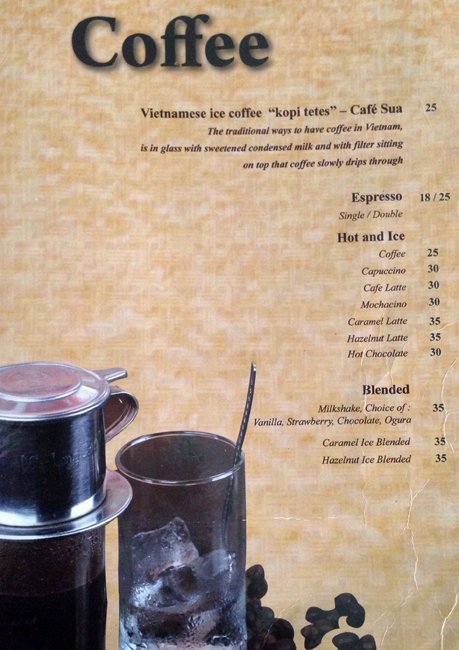The image depicts a well-used and slightly crumpled menu from a coffee shop, set against a light tan, splattered background. At the very top, prominently displayed in large black letters, is the word "Coffee." Beneath this header, the menu lists various coffee options and their prices in brown lettering. Key offerings include Vietnamese Ice Coffee, highlighting traditional preparation methods with sweetened condensed milk and a drip filter, alongside more familiar choices such as Espresso (available as single or double shots), Hot and Iced Coffee, Cappuccino, Cafe Latte, Mochaccino, Caramel Latte, Hazelnut Latte, and Hot Chocolate. Additionally, there are blended drink options like Milkshakes in Vanilla, Strawberry, Chocolate, and Agoura flavors, as well as Caramel and Hazelnut Ice Blended beverages. The lower left corner of the menu features an image of a coffee pot, a glass with ice, a spoon, and some scattered coffee beans, enhancing the coffee-centric theme.